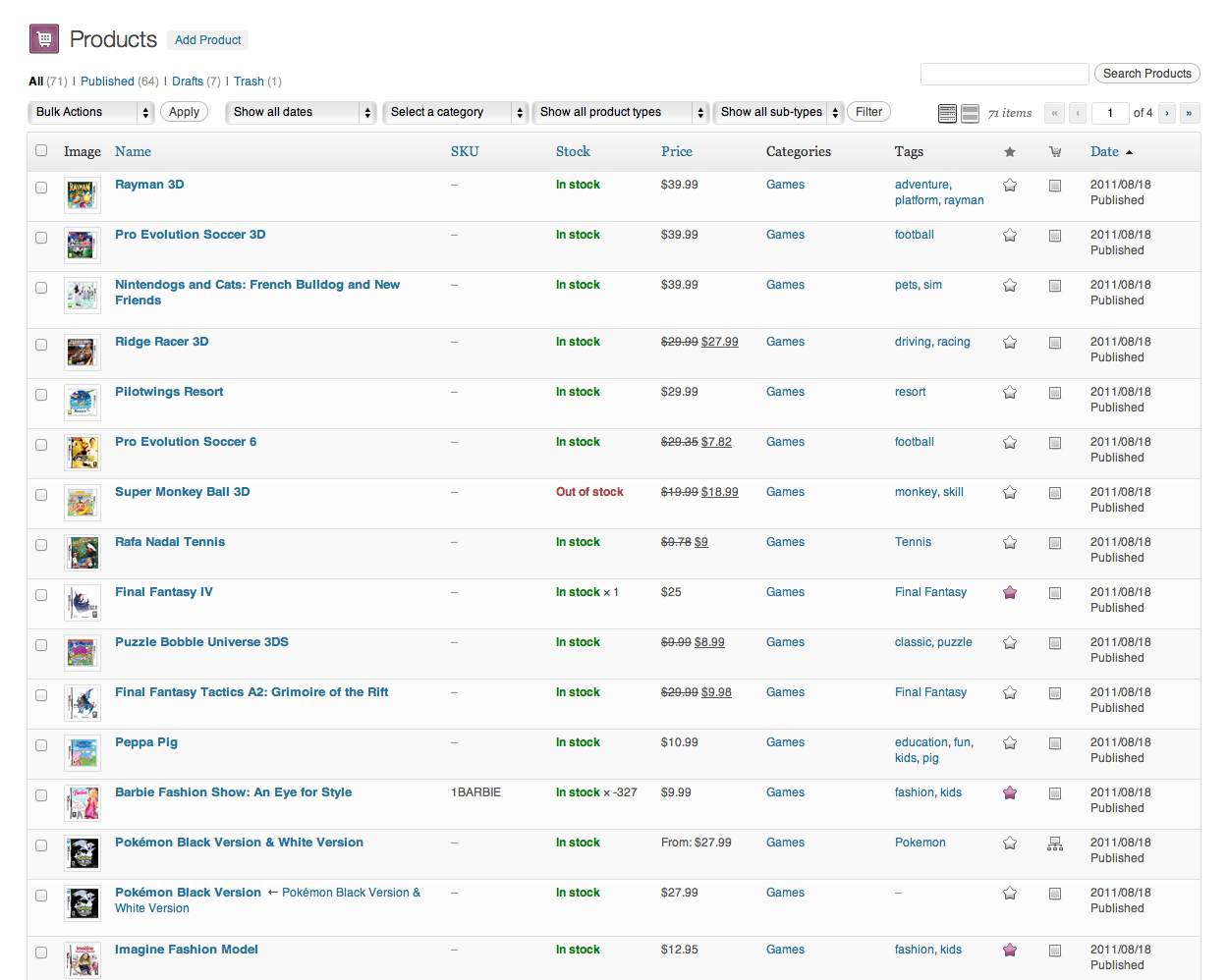**Screenshot of Shopping Cart and Product Management Page**

This image is a detailed screenshot of a shopping cart or product management interface. At the top, there is a shopping cart icon followed by a menu with options such as 'Products', 'Add Product', and quick filters like 'All (71)', 'Published (64)', 'Drafts (7)', and 'Trash (1)'. To the right is a search box labeled 'Search products'.

Below this, a banner with various filtering options is displayed, including 'Bulk actions' with an 'Apply' button, 'Show all dates', 'Select a category', 'Show all product types', 'Show all subtypes', and a 'Filter' button. This banner also contains navigation icons and back and forward buttons, indicating the current view is page 1 of 4.

The data table lists products with columns for Image, Name, SKU, Stock, Price, Categories, Tags, a Star (likely for featured products), a shopping cart icon, and Date. The table appears to be sorted by Date, as indicated by a small arrow next to the Date header.

**Product List with Details:**

1. **Rayman 3D**
   - Stock: In Stock
   - Price: $39.99
   - Categories: Games, Adventure, Platform
   - Date: 2011-08-18
   - Status: Published

2. **Pro Evolution Soccer 3D**
   - Stock: In Stock
   - Price: $39.99
   - Categories: Games, Football

3. **Nintendogs and Cats: French Bulldog and New Friends**
   - Stock: In Stock
   - Price: $39.99
   - Categories: Games, Pets, Sim

4. **Ridge Racer 3D**
   - Stock: In Stock (On Sale)
   - Original Price: $29.99
   - Sale Price: $27.99
   - Categories: Games, Driving, Racing

5. **Pilot Wings Resort**
   - Stock: In Stock
   - Price: $29.99
   - Categories: Games, Resort

6. **Pro Evolution Soccer 6**
   - Stock: In Stock (On Sale)
   - Original Price: $29.35
   - Sale Price: $7.82
   - Categories: Games, Football

7. **Super Monkey Ball 3D**
   - Stock: Out of Stock
   - Price: Original $19.99, Last $18.99
   - Categories: Games, Monkey, Skill

8. **Rafa Nadal Tennis**
   - Stock: In Stock (On Sale)
   - Original Price: $9.78
   - Sale Price: $9.00
   - Categories: Games, Tennis

9. **Final Fantasy 4**
   - Stock: In Stock (1 Unit)
   - Price: $25.00
   - Categories: Games, Final Fantasy

10. **Puzzle Bobble Universe 3DS**
    - Stock: In Stock (On Sale)
    - Original Price: $9.99
    - Sale Price: $8.99
    - Categories: Games, Classic Puzzle

11. **Final Fantasy Tactics A2: Grimoire of the Rift**
    - Stock: In Stock (On Sale)
    - Original Price: $29.99
    - Sale Price: $9.98
    - Categories: Games, Final Fantasy

12. **Peppa Pig**
    - Stock: In Stock
    - Price: $10.99
    - Categories: Games, Education, Fun, Kids, Pig

13. **Barbie Fashion Show: Her Style**
    - Stock: Negative $3.27
    - Price: $9.99
    - Categories: Games, Fashion, Kids

14. **Pokemon Black Version and White Version**
    - Stock: In Stock
    - Price: $27.99
    - Categories: Games, Pokemon
   
15. **Imagine Fashion Model**
    - Stock: In Stock
    - Price: $12.95
    - Categories: Games, Fashion, Kids